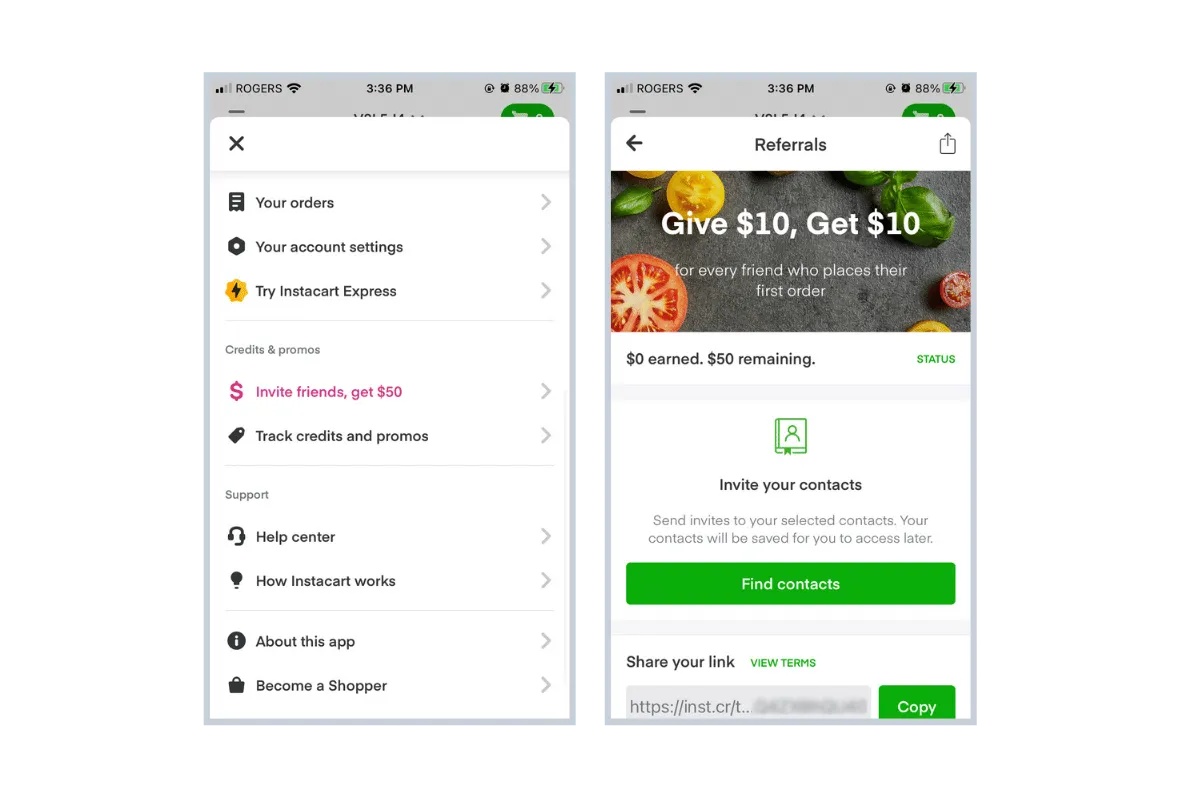The image contains two screenshots of a mobile application. 

### Left Screenshot:
This screen displays the main menu of an app against a white background with various options listed in black text, each followed by a right-facing caret mark on the right side:
1. **Your Orders**
2. **Your Account Settings**
3. **Try Instacart Express**

Separating these sections is a thin, black horizontal line. The subsequent options appear in gray and pink text:
1. **Credits and Promo** (gray) 
2. **Invite Friends, Get $50** (pink) 
3. **Track Credits and Promos** (black)

Each of these options similarly includes a right-facing caret mark. Following another thin black separator, additional options are provided in gray and black text:
1. **Support** (gray) 
2. **Help Center**
3. **How Instacart Works**
4. **About This App**
5. **Become a Shopper**

Each of these entries also displays a right-facing caret mark.

### Right Screenshot:
This screen highlights the "Referrals" section of the app. At the top is the header "Referrals." Below this, a header image depicts a black or gray table with various cut-up fruits and vegetables, including a tomato, green leaves, and a yellow fruit (possibly a lemon). Overlaid on this image in white text is the offer: "Give $10, Get $10 for every friend who places their first order."

Below the image, against a white background, black text states:
- **$0 Earned, $50 Remaining** 
- **Status** in green

Next, a contact icon is displayed with the text "Invite Your Contacts" beneath it. In gray text, it reads: "Send invites to your selected contacts. Your contacts will be saved for you to access later."

A green button follows, labeled "Find Contacts" in white text. Below this, the user is prompted to "Share Your Link," highlighted in black text, followed by a box containing a web address or link. To the right of this box is another green button with the label "Copy" in white text.